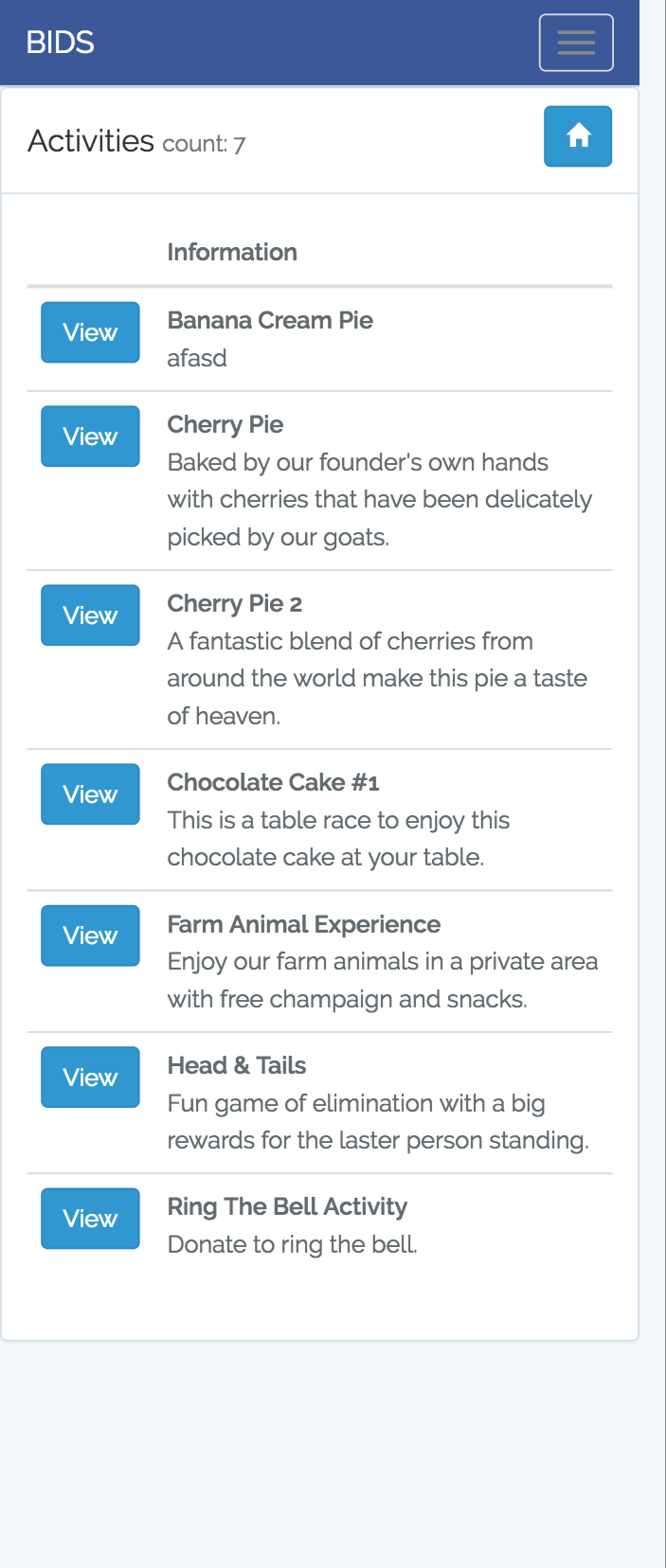The image is a vertical screenshot showcasing a mobile-optimized webpage from the BIDS platform. At the very top, a thin navy blue bar spans the width of the screen. On the left end of this bar, the word "BIDS" is displayed in white, uppercase letters. The top right corner features a menu icon, represented by three horizontal bars stacked vertically within a white square.

Below the blue bar, the word "Activities" is prominently displayed, followed by the number seven, indicating the count of activities listed. To the right of this text is a small blue button with a house icon.

The main content of the page lists several activities, each accompanied by a blue rectangular button labeled "View" in white text. The activities are as follows:
1. **Banana Cream Pie, A-F-A-S-T**
2. **Cherry Pie**: Baked by our founder’s own hands with cherries delicately picked by our goats. 
3. **Cherry Pie Too**: A fantastic blend of cherries from around the world, making this pie a taste of heaven.
4. **Chocolate Cake Number One**: Participate in a table race to enjoy this chocolate cake at your table.
5. **Farm Animal Experience**: Enjoy our farm animals in a private area with complimentary champagne and snacks.
6. **Head and Tails**: A fun elimination game with big rewards for the last person standing.
7. **Ring the Bell Activity**: Donate to ring the bell.

Each activity description is brief yet enticing, offering unique experiences or delicious treats.